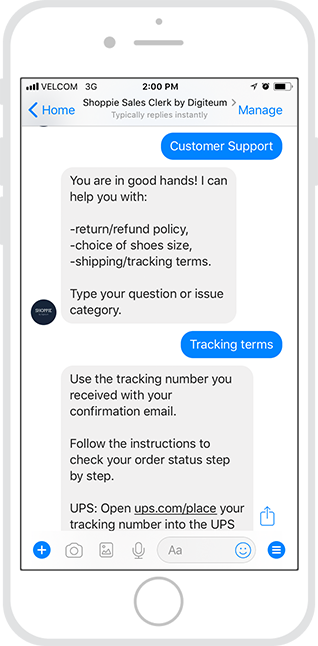The image features a digital rendering of an older model white iPhone, characterized by the prominent home button at the bottom of the device. The phone's screen displays a screenshot of a conversation from iMessages, which appears to have been digitally added to emphasize the interaction. The top left of the screen shows the signal as "Velcom 3G" and includes the time and battery status, reflecting the interface of a previous iPhone generation.

The displayed message appears to be from a service named "Shopee Sales Clerk by Digitium," which claims to offer prompt replies, suggesting it might be a customer service or support bot. The interface shows text options with "Home" on the top left and "Manage" on the top right.

The conversation reads:

"Customer Support: You’re in good hands. I can help you with:
- Return/Refund Policy
- Choice of Shoe Size
- Shipping/Tracking Terms

Type your question or issue category."

The customer replies with "Tracking Terms," to which the support responds:

"Use the tracking number you received in your confirmation email: UPS ###."

The image seems to serve as an illustration of customer service capabilities rather than depicting a genuine conversation, likely intended to showcase the quality of service provided by the entity.